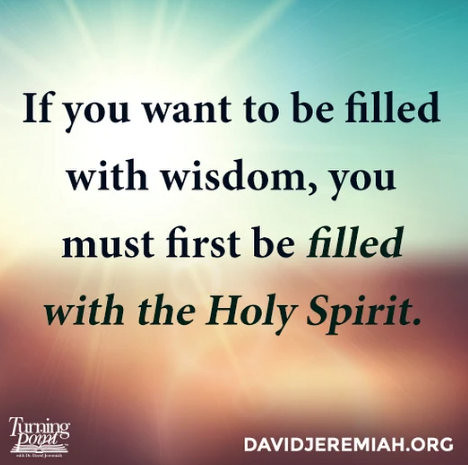The image features a square graphic centered on a blurred horizon background that is divided into a brownish bottom half and a blue upper half. A radiating sun in the left mid-section emits bright light and rays, enhancing the serene atmosphere. In the center of the image, black text boldly states, "If you want to be filled with wisdom, you must first be filled with the Holy Spirit." Positioned in the lower left corner, a white logo reads "Turning Point" accompanied by an illustration of a book, while the bottom right corner displays the URL "davidjeremiah.org" in white text. The overall design emphasizes a contemplative message set against a tranquil, diffused landscape.